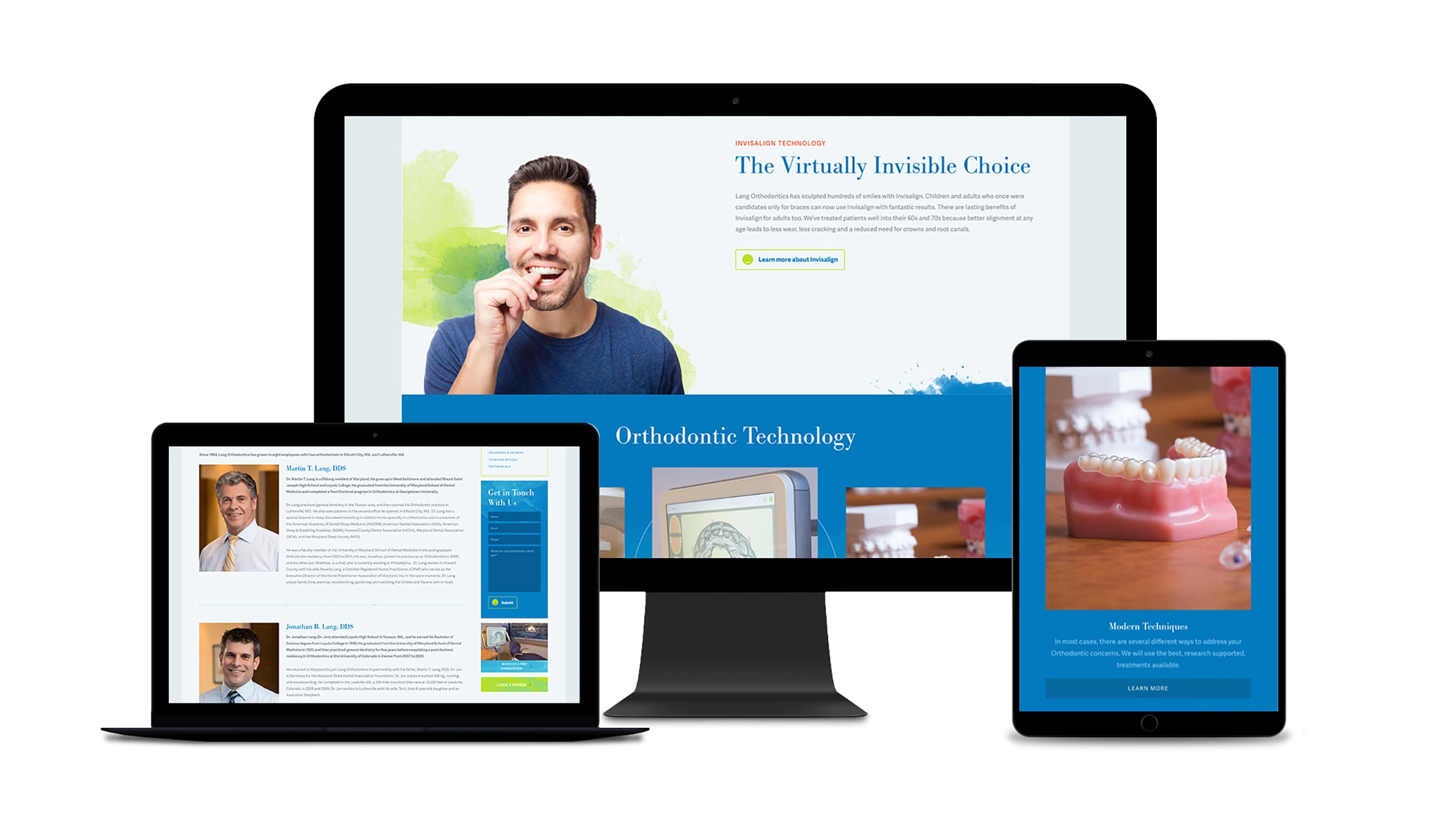Screenshot of a digital workspace showcasing three devices: a computer monitor, a laptop, and a tablet. The computer monitor displays an advertisement for Invisalign, highlighting its "virtually invisible choice" for orthodontic technology, accompanied by an image of a man in a blue shirt inserting Invisalign aligners with a beaming smile. The laptop screen features several photographs of dental professionals, likely orthodontists, sharing their insights and reviews on Invisalign. Meanwhile, the tablet screen presents an image of a lower gum set of dentures, with a plaster cast of a lower set of teeth positioned in the background.